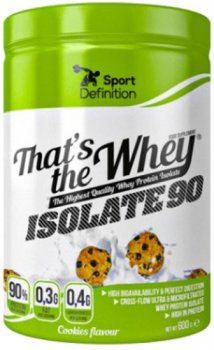A cylindrical lime green bottle of protein powder is prominently displayed. The bottle features a large white label that wraps around its middle, with a striking design that includes the brand name "That's The Whey" in bold lettering. The word "Whey" is especially notable, with an elongated 'Y' that underlines the phrase "That's The," where it proudly proclaims "The Highest Quality Whey Protein." Although some text is difficult to discern, the label also mentions "Isolated 90" and is adorned with comprehensive calorie and nutrition information. The product is identified as being by "Sports Definition." The package art includes an image of cookies being splashed into milk, suggesting a cookies and cream flavor. This eye-catching design clearly communicates the premium quality and flavor of the protein powder inside.